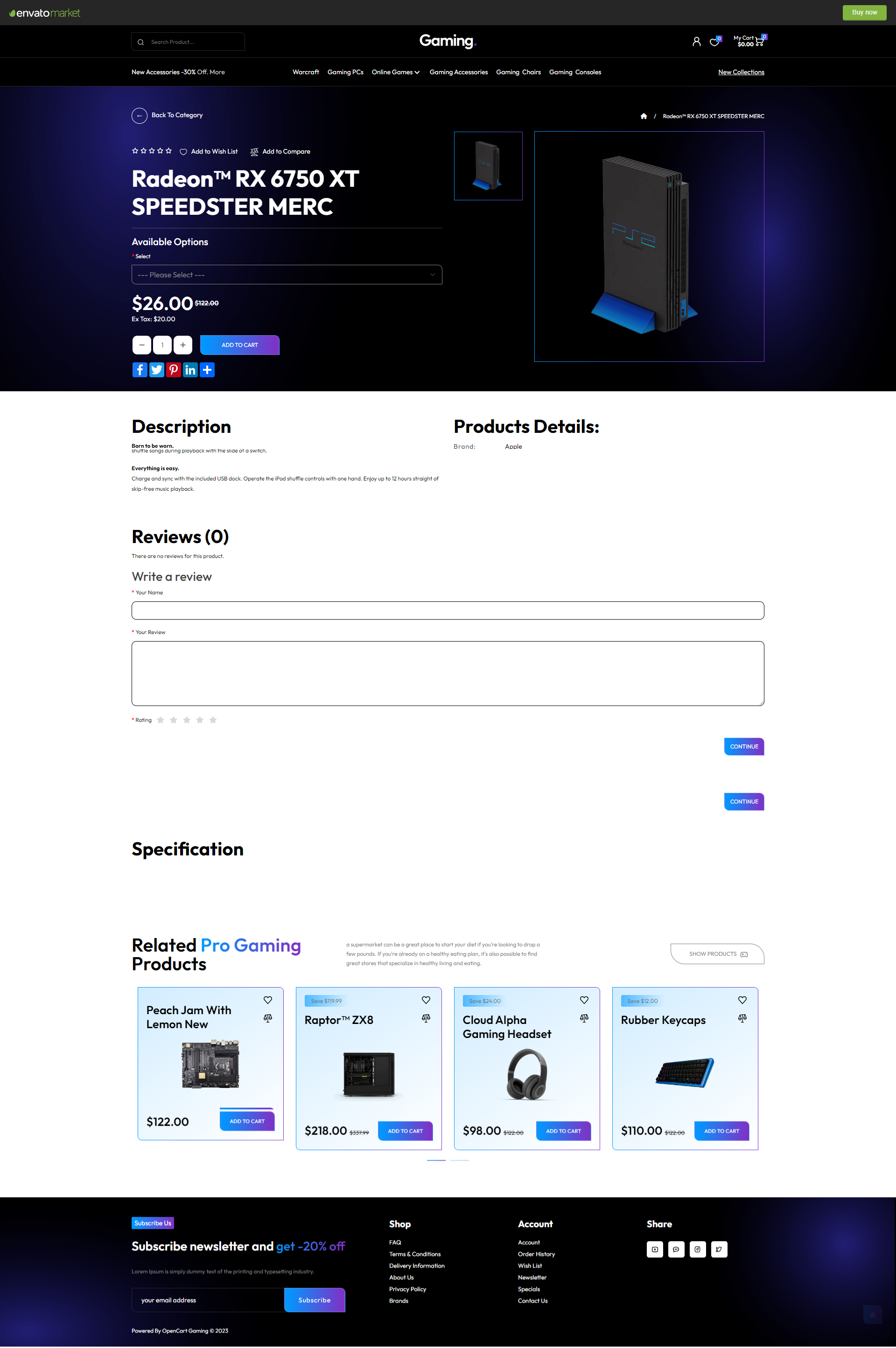In this image, there is a clean white background. At the top of the image, a large black box prominently displays the word "Gaming" in white font. Below this, a series of small, differently categorized headings stretch across the top.

Central to the image is the text "Radeon RX 6750 XT Speedster Merc," followed by a price tag of "$26" and a conspicuous blue button. Social media icons, including Facebook, are arrayed in the same section against a dark blue backdrop. An additional small box features an image of the Radeon RX 6750 XT Speedster Merc, which is black with blue accents at the bottom. Below it is a larger picture of the product with a blue background and white text overlay.

Further down, the white background resumes, hosting detailed descriptions and product details highlighted in blue. The section also includes user reviews, tallying up to 10, with an invitation to "Write a Review" accompanied by a relevant text box. Following this, another large white box appears, featuring two small blue buttons labeled "Specification" and "Related Products."

The image continues to showcase a "Pro Gaming" section, marked by a few blue lines, and next to it, a white square with blue text. Further down, four small blue squares exhibit different products, each with a blue button at the bottom right corner. Finally, the bottom of the image is anchored by a large black box, which includes a small blue button at the top, white text, and another blue button at the bottom. Adjacent to this are four small white boxes positioned on the right side of the black box.